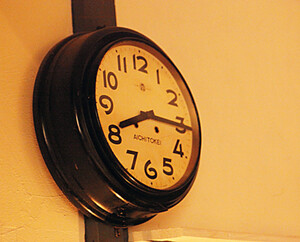The photograph captures a circular wall-mounted clock attached to a cream-colored wall, though the lighting in the room casts a yellowish tint over the scene. The clock's face, predominantly cream-colored with possible yellow accents, is encased in a black housing and mounted on a vertical metal beam that connects it to the wall. The clock’s face displays traditional black numerals from 1 to 12, each accompanied by a thick black line with thinner hash marks in between. The current time shown is a quarter past eight, with the hour hand just past the 8 and the minute hand on the 3. The clock lacks a second hand and has two small black holes between the hour and minute hands, likely for winding. An inscription, which is difficult to read due to the angle, appears between the numbers 5, 6, and 7, possibly spelling "A-C-H-I-T-O-K-E-I" in black. The overall setting suggests an indoor environment with dim, yellowish lighting, giving the clock a vintage feel.